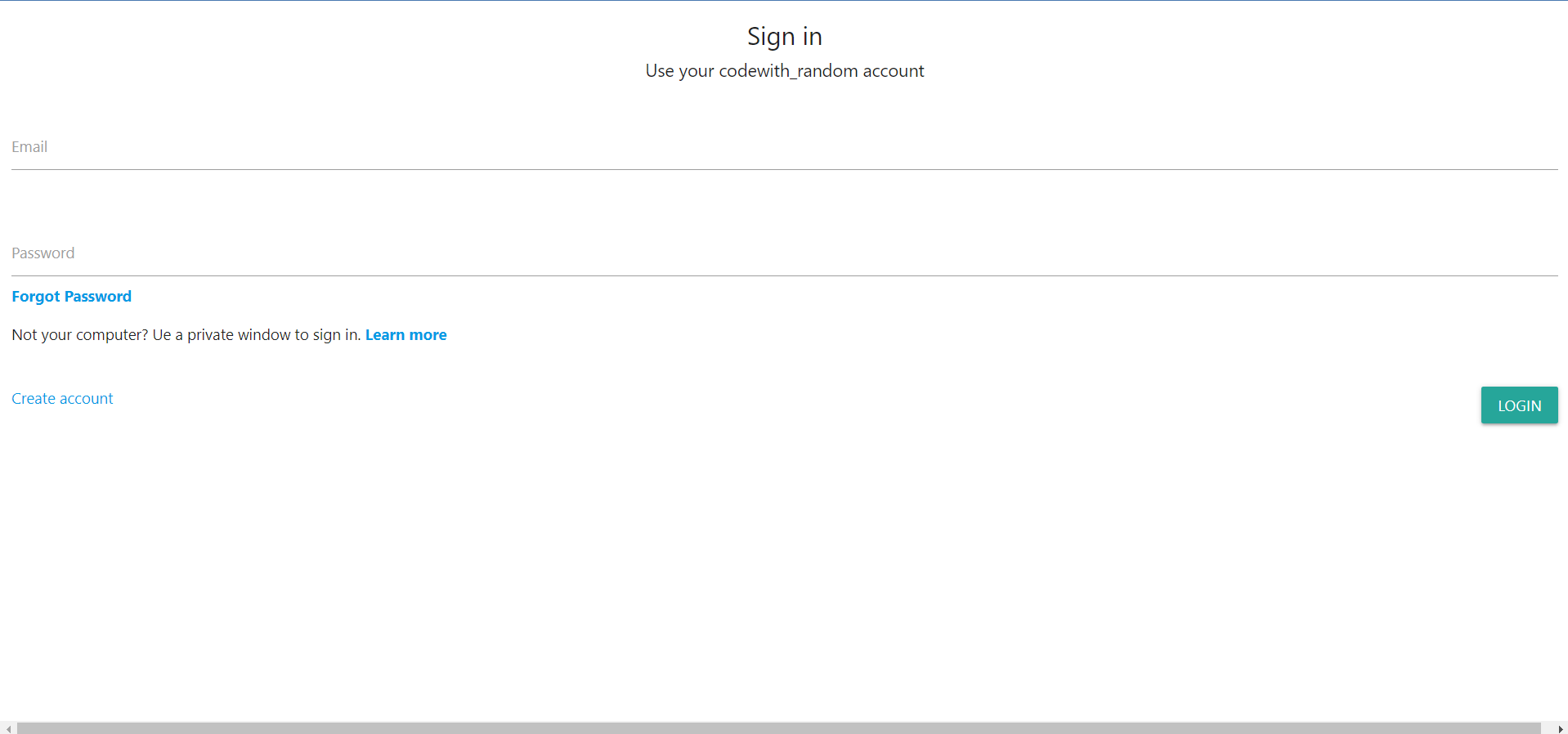The website features a predominantly white background with various colored fonts. At the top of the screen, there's a thin horizontal line stretching from one side to the other. The bottom of the screen includes a horizontal scrollbar for navigation if the content exceeds the visible area.

At the center of the page, a bold black font prominently displays "Sign In." Below that, non-bolded text reads "Use your code with _random_account." A long horizontal line spans the screen beneath this text. Following that, the form fields for "Email" and "Password" are presented in gray text, each with a horizontal line below it.

Underneath the password field, a bolded "Forgot password?" appears in bright blue, indicating a hyperlink. Further down, black text informs, "Not your computer? Use a private window to sign in," followed by another blue hyperlink stating "Learn more."

A lighter-shaded text suggests "Create account" towards the bottom. Lastly, on the left side of the screen, there is a small rectangular green button with "Login" written in white font.